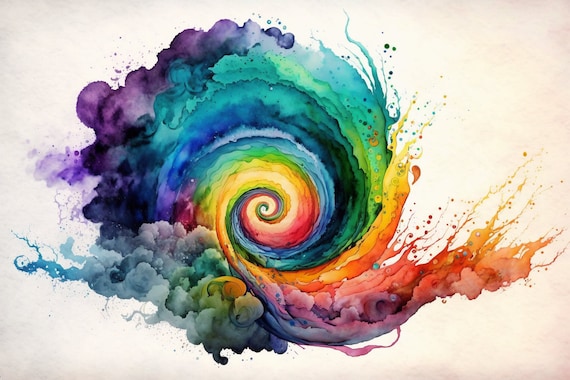The image depicts a colorful, spiral-shaped drawing at its center, resembling a snail shell or a cyclone, which gradually expands outward and transitions into cloud-like formations. The spiral starts with vibrant yellows, greens, and oranges at its core, and as it extends outward, it morphs through an array of colors, including shades of red, purple, blue, and yellow. The spiral is detailed with smooth gradients, where, for example, red fades into yellow and then back to red. Surrounding the central spiral, particularly on the bottom left, are cloud-shaped objects, as if the spiral is dispersing into wisps of clouds. The background of the image features a blend of pale purple on the left and pale pink on the right, though it mostly appears white, serving as a clean canvas for the vibrant colors. Additional splashes of color, including orange, pink, and purple, add dynamic elements to the scene, along with some paint splatters and water-like textures at the edges. The outer regions of the spiral also include hints of green, yellow, and blue, combining to create a lively and intricate composition.